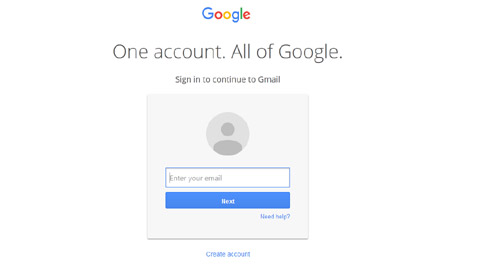A screenshot of a Google sign-in page is displayed, prominently featuring the Google logo at the top. Below the logo, the phrase "One account. All of Google." is clearly visible. The page instructs users to "Sign in to continue to Gmail."

There is an icon resembling a person's head, representing the user profile, next to a text input bar labeled "Enter your email." This input bar is highlighted by a rectangular outline, drawing attention to it. 

Beneath the email input bar is a large, striking blue button labeled "Next," which guides users to the next step in the sign-in process. 

Additionally, there are links for "Need help?" offering troubleshooting options, and "Create account" for users who do not yet have a Google account. 

The entire interface is designed with a light gray and white color scheme, maintaining a clean, minimalist look. The text "One account. All of Google" appears multiple times, emphasizing the unified access provided by a single Google account. The overall visual layout is simple and user-friendly, guiding users through the sign-in process seamlessly.